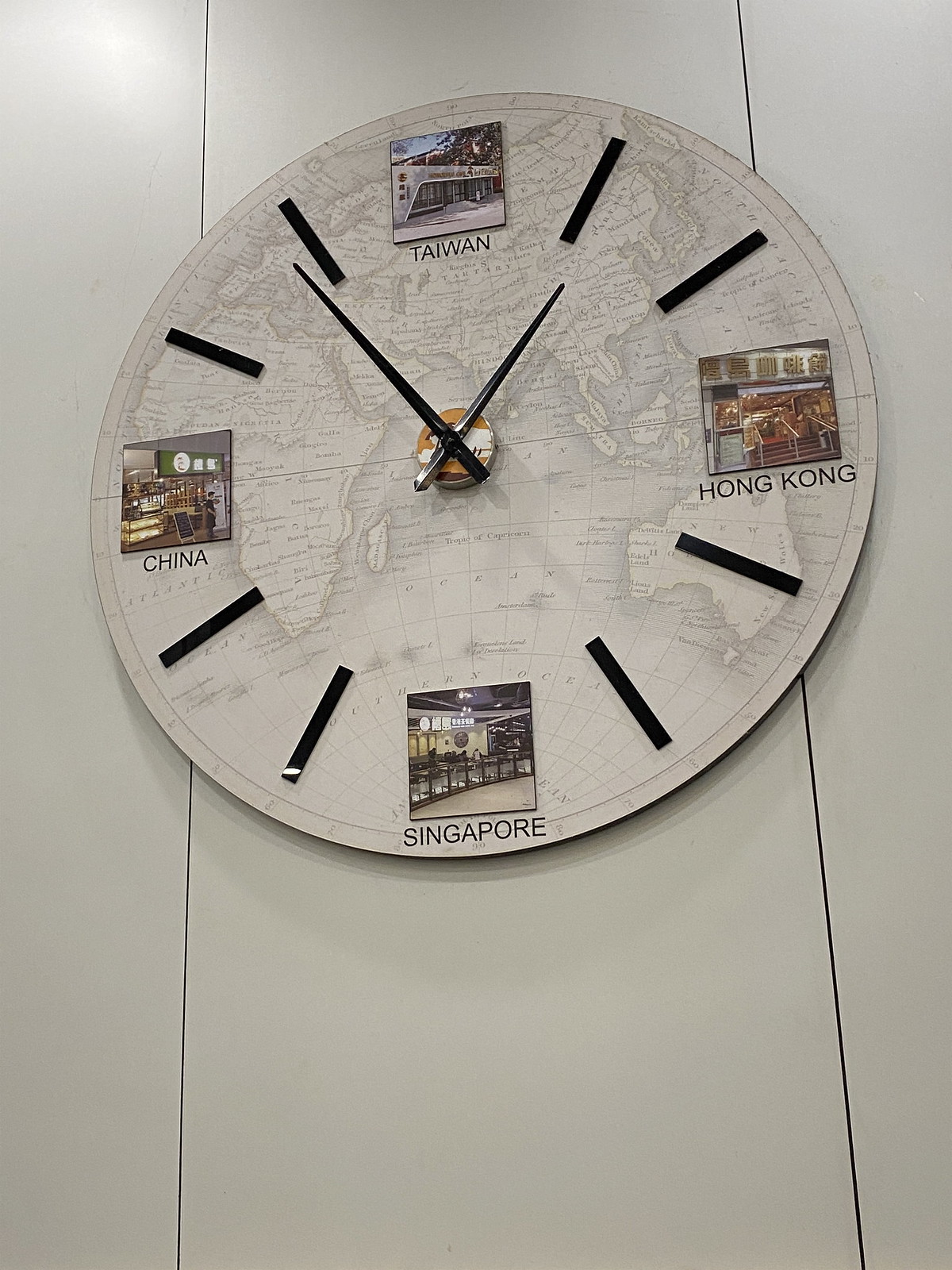The image features a distinctive wall clock mounted on an off-white wall with two thin black vertical seams running from top to bottom. Positioned centrally and at the top of the image, the clock spans both seams, interrupting their flow momentarily. The clock's earthy, tan-colored face resembles a globe, with a detailed map focus on Asia. 

At the 12 o'clock position, there is a small square inset labeled "Taiwan" with a representative image. Similarly, the 3 o'clock mark features "Hong Kong," 6 o'clock displays "Singapore," and the 9 o'clock spot highlights "China," each accompanied by small images embodying their respective regions. Instead of numbers, black lines indicate the hours between these key points. The clock hands, sharp and black, reminiscent of chopsticks, suggest an Asian theme. 

The time shown on the clock is approximately six minutes to two. The clock's backdrop portrays a detailed map with the center placed over the Indian Ocean, and the entire clock face integrates with the global motif, casting it possibly as a creative piece suitable for an office, hotel, or business setting with a focus on Asia.